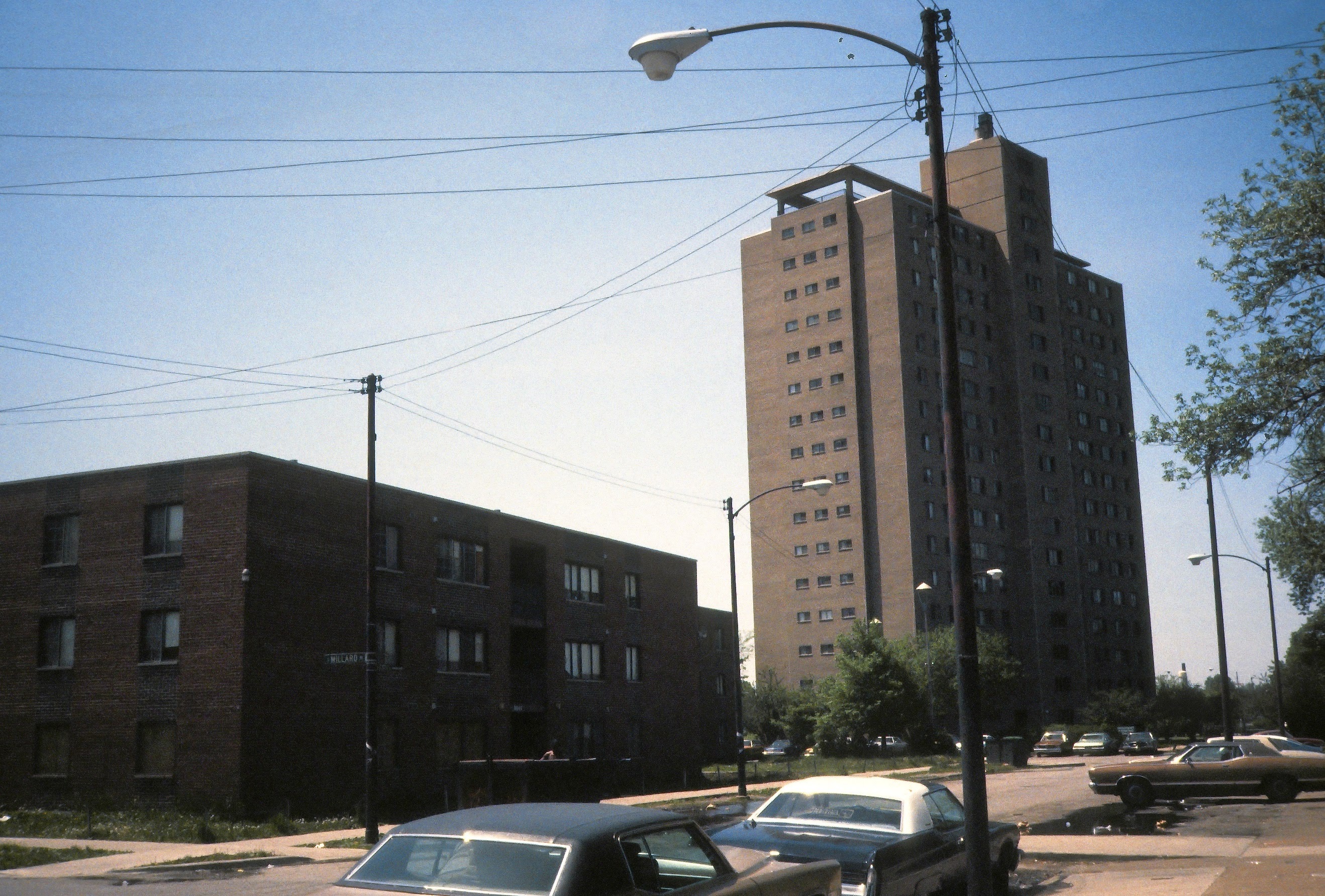The image depicts a city street scene from the 1970s or 1980s under a clear, gradient blue sky. Dominating the scene are two adjacent brown buildings. The larger building, appearing as a high-rise with approximately 15 to 16 floors, is lighter brown and features various sections, including a part that extends higher with possible deck areas on the roof. In front of it stands a smaller, three-story, darker brown building. The street in front of these buildings is devoid of people but populated with several cars, estimated around 15, representative of 1970s models. Among them, a brown car with a black roof, a blue car with a white roof, and another brown car perpendicular to the others are particularly noticeable. The scene is complemented by greenery, with at least two trees visible—one between the buildings and another on the right edge of the photo. Several street lamps and crisscrossing wires add to the urban setting, though no street signs or wording can be observed. The overall appearance suggests an older, possibly historical moment captured from several decades ago.